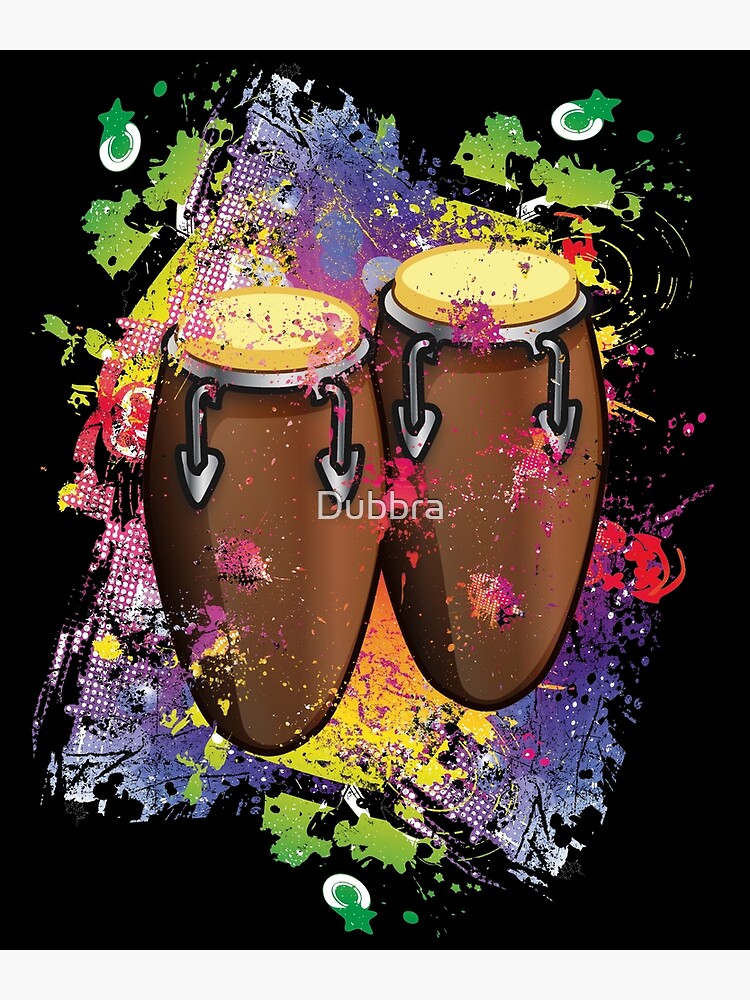This detailed digital painting showcases two large, tall hand drums, placed side by side, resembling oversized bongos. The drums feature a rich brown color with a yellow top, accented by a strip of silver at the bottom and secured with silver hooks. The background is a vibrant array of color splashes, including yellow, blue, green, white, orange, purple, and red, with pink and blue areas adorned with white polka dots. These colorful splatters and markings create a dynamic and lively backdrop, with additional designs of stars and circles dispersed throughout. The outer edges of the background transition into black, framing the central composition. Across the front middle of the image, the word "Dubbra," spelled D-U-B-B-R-A, is prominently displayed in whitish-gray letters. The overall artistic design evokes the rhythmic energy of playing hand drums, possibly African war drums, against a visually stimulating background.